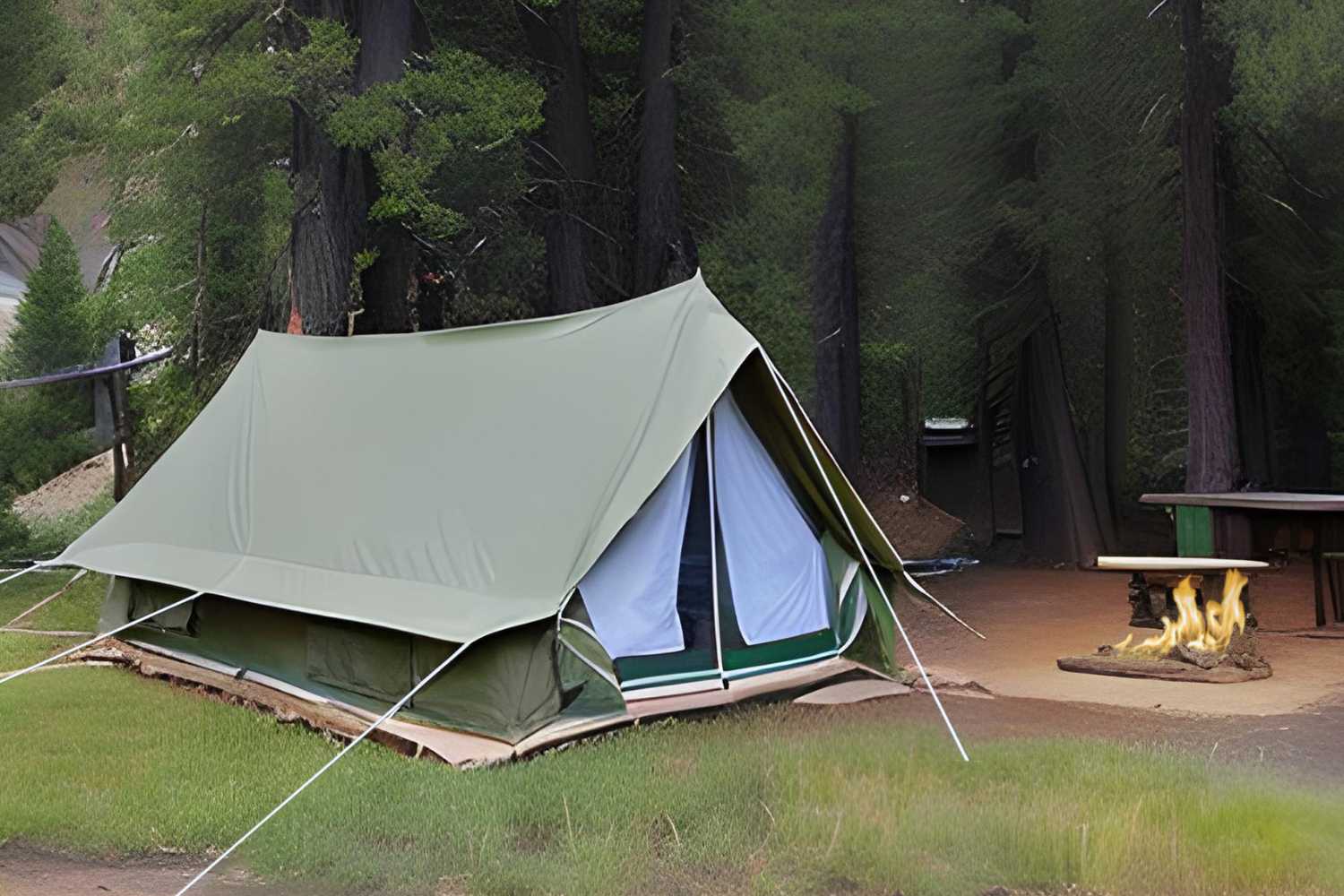This image, likely AI-generated due to its peculiar details, showcases a campsite set outdoors. Central to the scene is a large, green tent, possibly able to accommodate six people. The tent is secured with white bungee cords that stretch out to the sides, though they seem to vanish into the ground without visible stakes. The tent's entrance consists of two white panels bordered by blue-green fabric. Flanking the tent on the right is a burning campfire composed of several logs. Nearby, a picnic table is partially obscured. The backdrop reveals a collection of tall trees, including a distinct pine tree to the far left behind a mound of dirt. Oddly, a lone door stands amidst the forest, contributing to the surreal atmosphere. The ground is covered with sparse, seemingly artificial grass, and the tent is set atop what appears to be an arrangement of cardboard and wooden pallets.